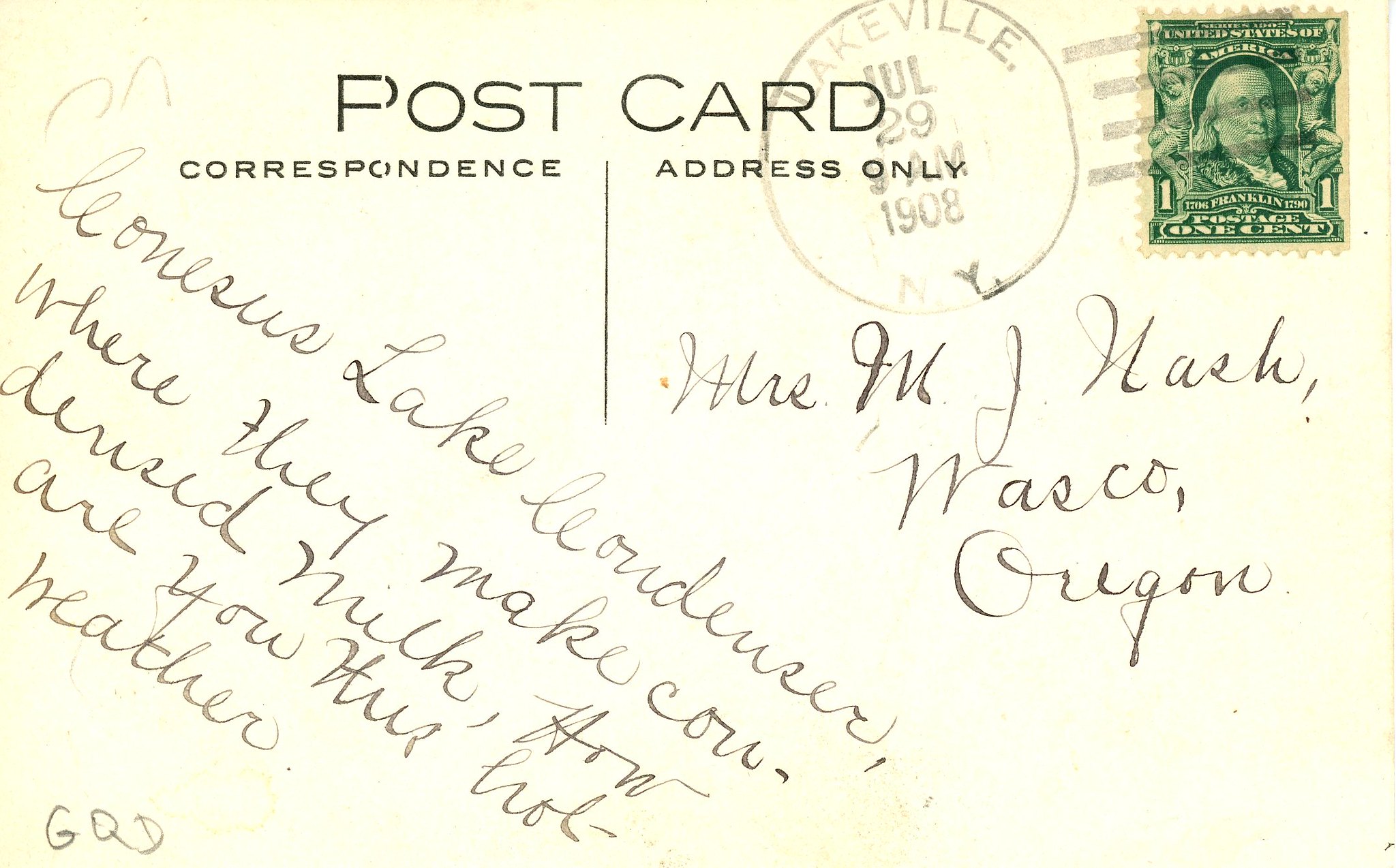This image depicts an old, horizontally aligned rectangular postcard with a vintage appearance. The postcard, predominantly beige with some light brown discoloration around the edges, is adorned with a green Benjamin Franklin one-cent postage stamp in the upper right corner. The stamp is marked with a postmark that reads "Lakeville, July 29, 1908." Bold black lettering at the top of the postcard announces "Postcard," with the phrases "Correspondence" and "Address only" situated below it. Handwritten in cursive on the left side of the postcard is a note that mentions "Leonisys Lake" and "Lord D'Azur, where they make condensed milk," followed by an incomplete and partially illegible message that starts with "How are you this hot weather?" and ends with "Heather" or initials "G-O-D." On the right side, the postcard is addressed to a Mrs. M. J. Nash of Wasco, Oregon. Despite the wear and tear of time, the sentiments and details preserved on this postcard provide a fascinating glimpse into early 20th-century correspondence.